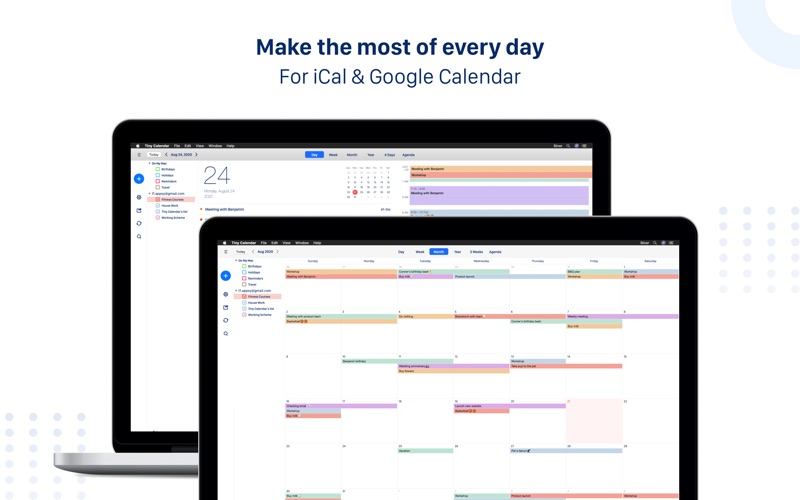Screenshot of an advertisement promoting calendar apps. The background is white and the image is in landscape orientation. Centrally featured are two stylized laptop screens with black outlines, each displaying a different type of calendar. The front screen shows a detailed calendar with color-coded activities; different colors seem to correspond to various activities, represented by small stripes on the days. For instance, one day includes stripes of red, lavender, and light blue, while other days show fewer or no stripes, indicating a less busy schedule. The background laptop showcases a thumbnail view of a monthly calendar, with a noticeable red dot on one of the days, possibly highlighting a specific date for further details. At the top of the webpage, in bold, dark blue text, is the phrase "Make the most of every day," followed by a smaller subheading that states "for iCal and Google Calendar."